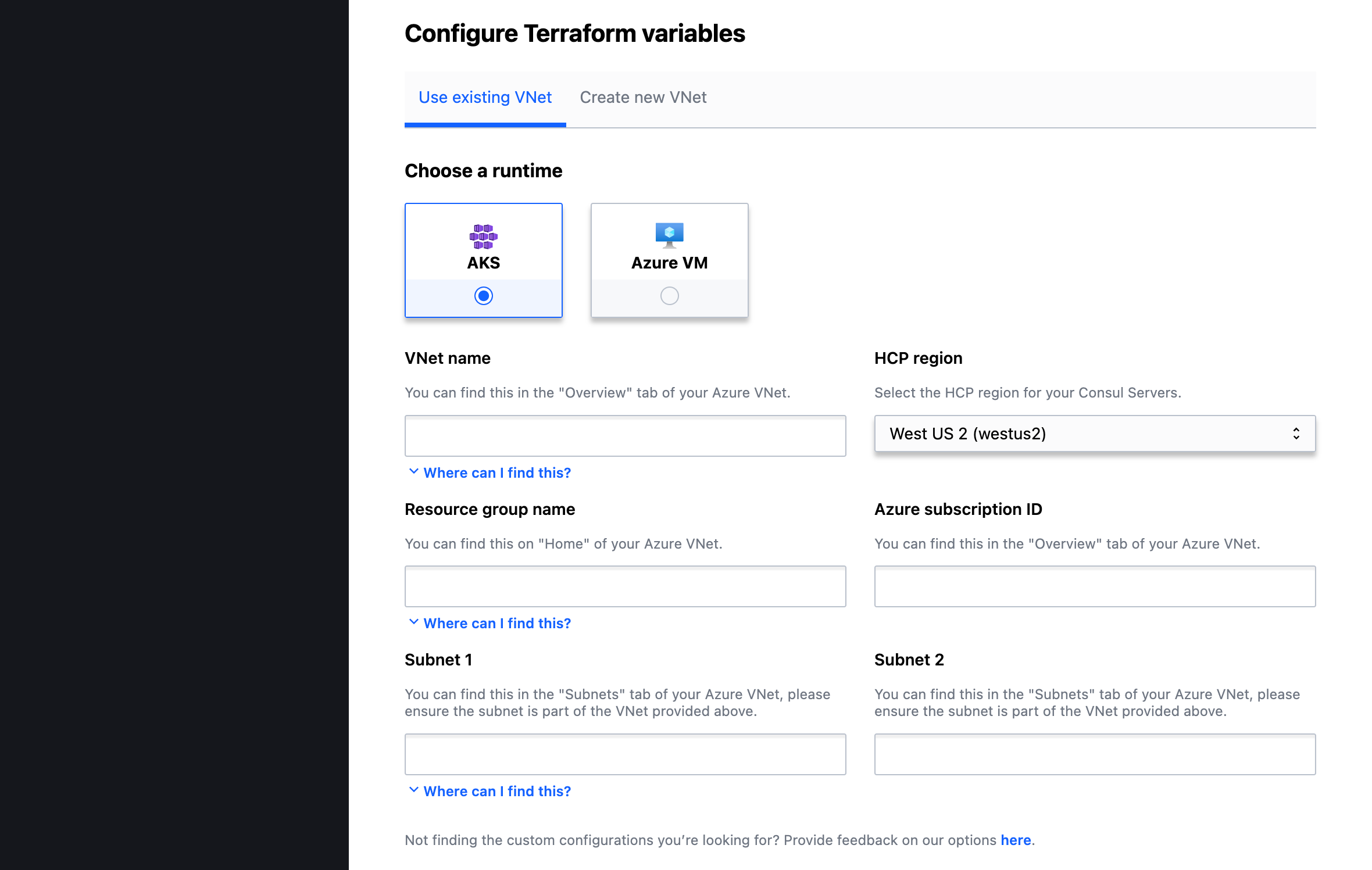The image depicts a website interface focused on configuring Terraform variables. 

A large, vertical black bar occupies the left side of the display without any text. Adjacent to this, the header reads "Configure Terraform Variables" in bold, dark black text. Below this header is a search bar. 

The section beneath the search bar offers two options: "Use Existing VNet," highlighted in blue with a corresponding blue bar underneath it, and "Create New VNet," which is in gray text. 

Further down, the site instructs users to "Resume a Runtime." There are two selectable boxes displayed. The first box is labeled "AKS" and features a filled blue circle with purple circles resembling grapes positioned above it. Next to this is another option, "Azure VM," depicted by an icon of a computer with a blue screen and an empty circle beneath it.

Following these options, the site provides input fields for "VNet Name" and "ACP Region," each accompanied by long text boxes for user input. A highlighted blue text link, "Where can I find this?" is available to guide users.

Below, there are fields for "Resource Group Name" and "Azure Subscription ID," both of which also feature text boxes for data entry and another "Where can I find this?" blue clickable link.

The form ends with inputs for "Subnet 1" and "Subnet 2," and again a blue link reads "Where can I find this?" It concludes with a note: "You can find this in the subnets tab on your Azure VNet. Please ensure the subnet is part of the VNet provided here."

Finally, a prompt at the bottom states, "Not finding the custom configurations you're looking for? Provide feedback on our options here," with the clickable feedback link highlighted in blue.